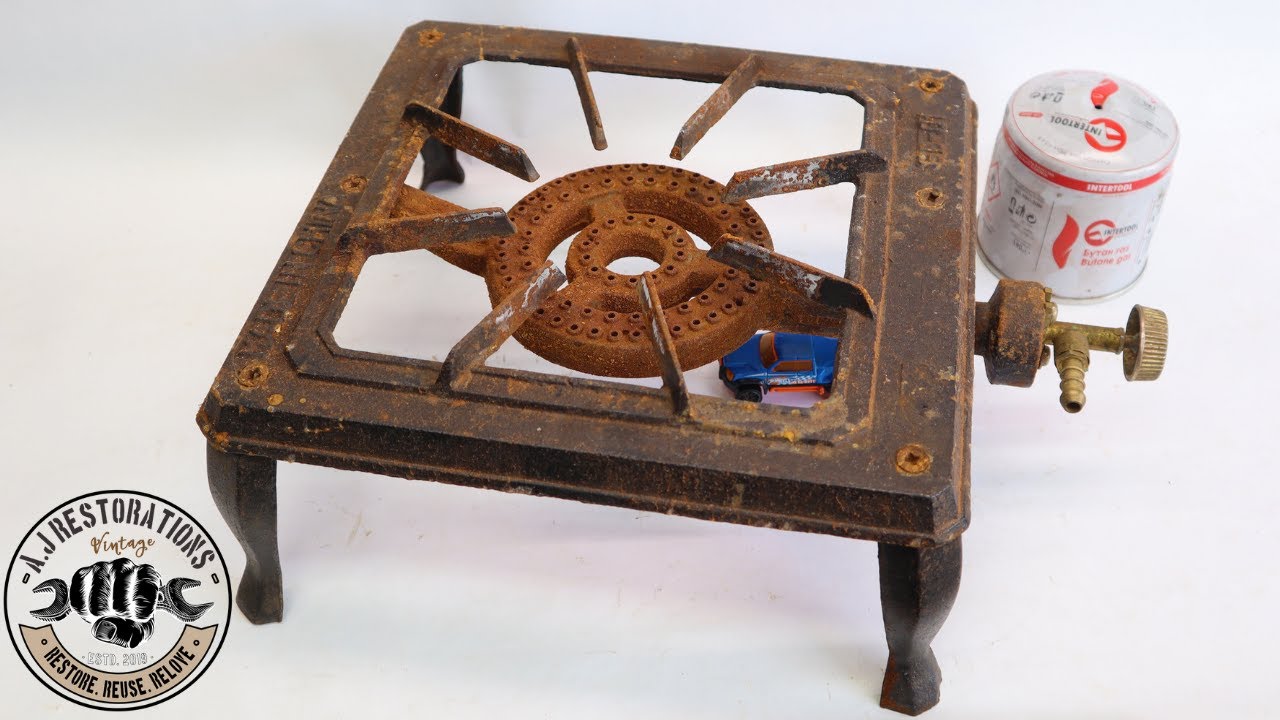The image features an old, rusted, portable gas stove, reminiscent of vintage camping equipment. The stove is square-shaped, elevated by four legs, and has a circular burner in the middle with nine prongs for supporting cookware. To the right of the burner is a gas nozzle meant for attaching a fuel canister. Nearby, in the upper right corner, there is a modern-looking, white propane container with red lettering, potentially indicating fuel for the stove.

Prominently placed in the bottom left corner is a black circle containing the logo for AJ Restorations. Inside the circle, the text reads "AJ Restorations, Vintage, Restore, Reuse, Relove," accompanied by an image of a black fist gripping a wrench, symbolizing the restoration process. Underneath the burner, there seems to be a blue toy car, though details are unclear. The overall scene suggests an effort to restore or repurpose the old gas stove, aligning with the ethos of AJ Restorations.